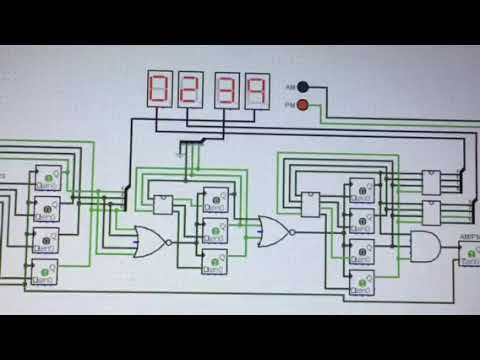The image showcases a rectangular, horizontally-aligned chart on a white background. The chart is bordered by thick black lines at the top and bottom. At the top, four black boxes house red digital numbers displaying "0239." To the right of these numbers, there is a black circle with a red circle located beneath it. The chart is covered in a complex array of green and black lines and dots that branch off in various directions, resembling an electrical or circuit diagram. This network of lines connects multiple black-outlined square boxes, each featuring a white center and small green LED lights. The boxes are arranged in a vertical formation: four on the left, three in the middle, four again on the right, and a single box on the far right. The lines and boxes create a detailed pattern, giving the impression of an intricate, possibly electronic, system diagram.